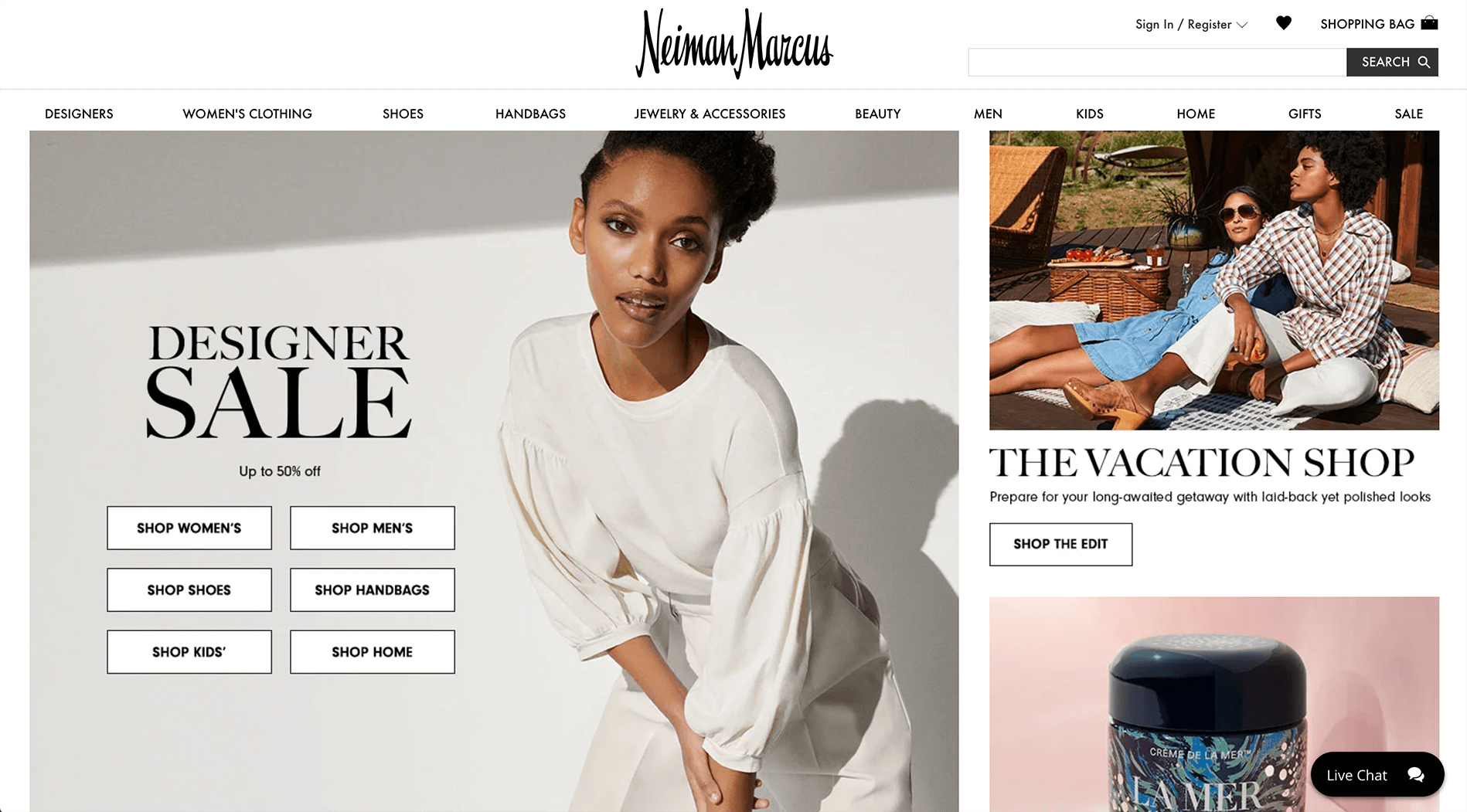The displayed image features a website layout that is approximately twice as wide as it is tall. At the top-most section, the background is pristine white, showcasing the elegant logo of Neiman Marcus in refined black lettering. To the right of the logo, there is a functional search bar with a black 'SEARCH' button to its right, featuring the word "SEARCH" in white, uppercase letters and accompanied by a white magnifying glass icon.

Above the search bar, you will find the sign-in and registration options, indicated by the text "SIGN IN / REGISTER" followed by a downward-facing arrow, all in black. A heart icon, filled with black, is situated next to it. Further to the right, the phrase "SHOPPING BAG" is prominently displayed in uppercase letters alongside a corresponding icon.

Beneath this header section, a horizontal menu in bold, capitalized black letters offers various categories: DESIGNS, WOMEN'S CLOTHING, SHOES, HANDBAGS, JEWELRY & ACCESSORIES, BEAUTY, MEN, KIDS, HOME, GIFTS, and SALE.

Dominating the left two-thirds of the webpage is a main banner. This banner features a young black woman dressed entirely in white. She is leaning forward, positioning herself diagonally towards approximately 6:30 or 7 o'clock on a clock face, with her head angled to the left, looking directly at the viewer. Positioned to her left, text in black declares "DESIGNER SALE," with additional text beneath proclaiming "UP TO 50% OFF." Six buttons, arranged in a grid of two across and three down, are displayed below this announcement. These buttons are white with black text, completing the cohesive and stylish presentation of the webpage.